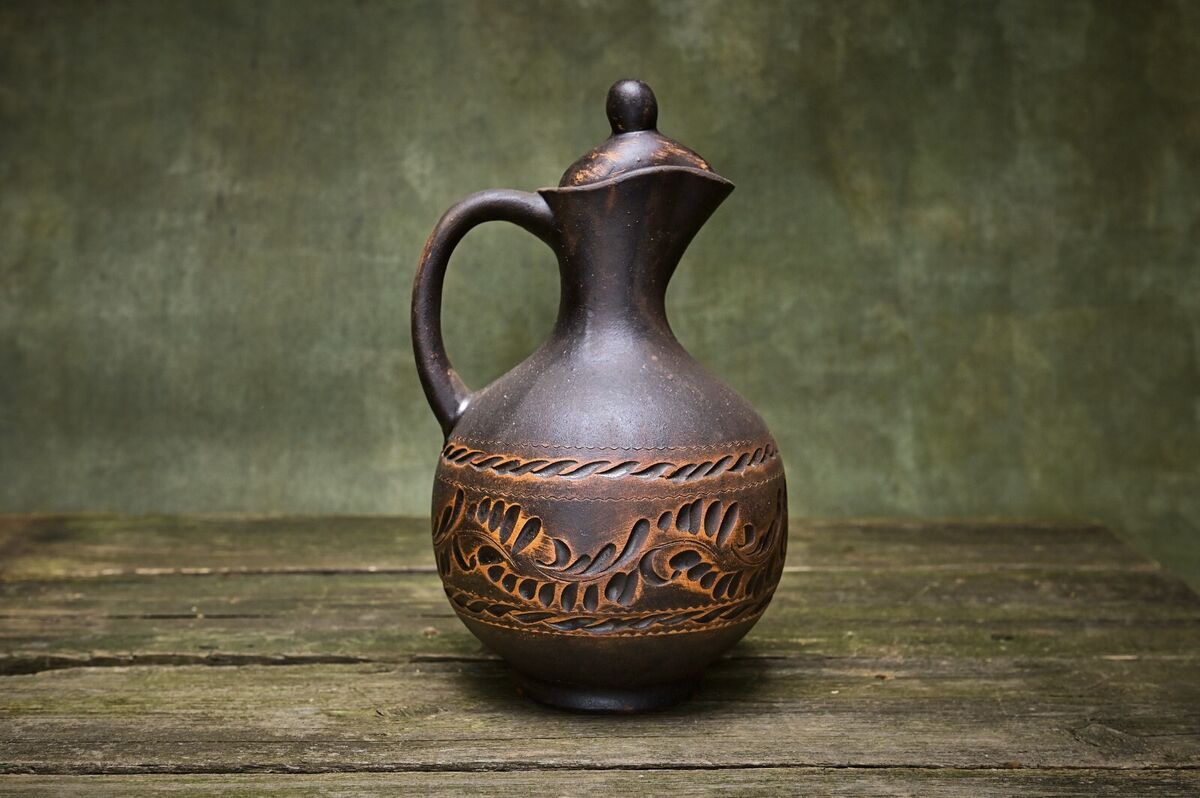The color photograph captures a meticulously detailed, computer-generated image of an earthenware urn designed for holding liquids, perhaps wine or water. The urn, crafted to resemble dark brown or almost black ceramic, features an intricate pattern of light brown oak leaves and flowers circling around its center. It possesses a gracefully curved handle on the left side and a generously wide base that tapers into a slender neck, before flaring out to form a top pour spout. The lid, topped with a small knob handle, is fitted securely into the opening at the top. This beautifully textured urn rests on a weathered, brown plank wooden table, which appears to be adorned with patches of moss, suggesting age and natural wear. The backdrop is a greenish wall, possibly concrete, under a lighting that casts subtle shadows and highlights, enhancing the urn's vintage yet newly created aesthetic.